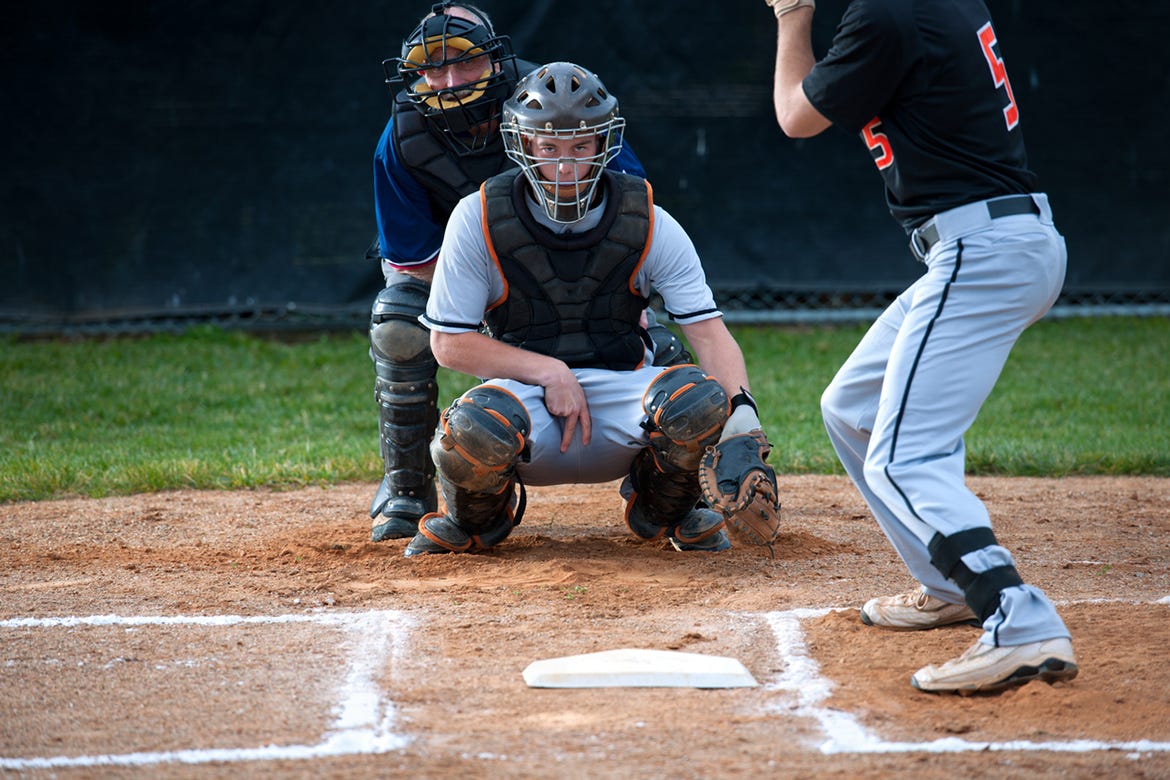This photograph captures a tense moment during a daytime baseball game from the pitcher's mound perspective. The rectangular image, about five inches wide and three inches high, prominently features the batter, catcher, and umpire in a rich, detailed setting. The bottom third of the image shows reddish-brown dirt with white chalk lines outlining the batter's box, and a white home plate centered within the frame.

In the right batter's box, poised and ready to swing, stands a batter. He’s equipped with white cleats, gray pants with a black stripe, and a very dark jersey emblazoned with the red number 5. His black belt and leg protector add to his readiness. The batter holds his bat back, his left foot lifted slightly off the ground, signaling his preparedness for the pitch.

In front of the batter, the catcher is squatted down in a vigilant stance. He wears gray pants with black stripes that match the batter's, and a lighter jersey underneath his chest protector. His protective gear includes a helmet and leg guards. His right hand extends between his legs, displaying a two-finger signal upside down – a directive to the pitcher. His left hand, encased in a mitt, rests beside his left leg, grounding him in position. The catcher, of Caucasian descent, stares ahead with focused determination.

Directly behind the catcher stands the umpire, partially emerging over the catcher’s right shoulder. Dressed in a very dark shirt and sporting protective leg guards and a head protector, the umpire diligently observes the unfolding action. The background transitions from the green grass of the outfield to a black tarp designed to catch stray balls, completing the vivid and detailed tableau of this crucial moment on the baseball field.